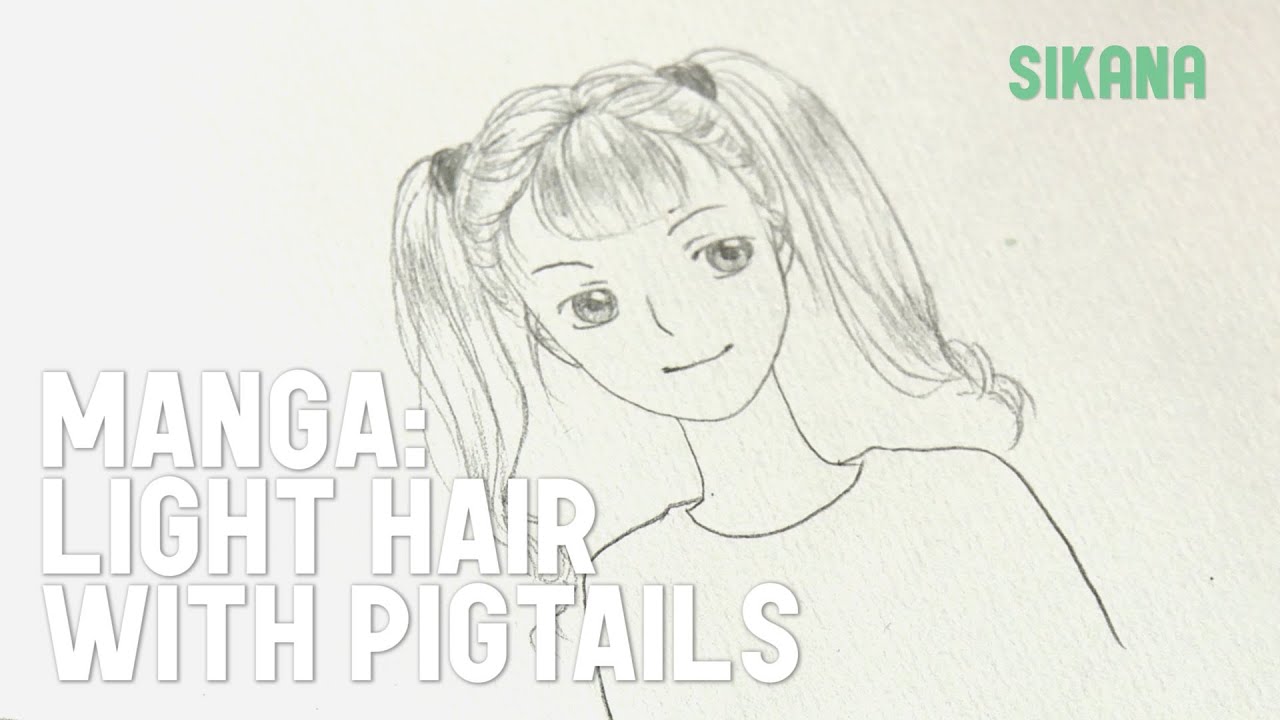The image is a pencil sketch of a little girl in a Japanese anime style, rendered on rough, textured sketchbook paper. The girl has shoulder-length hair styled into pigtails with black bands, a narrow face, and large, expressive anime-style eyes, eyebrows, and a mouth. In the top right corner, "Sakana" is written in green block text. On the lower left side, prominent white text with a gray outline reads: "MANGA: Light Hair With Pigtails." The sketch appears monochromatic, emphasizing shades of black and white. The overall composition suggests it might be intended as a YouTube thumbnail.